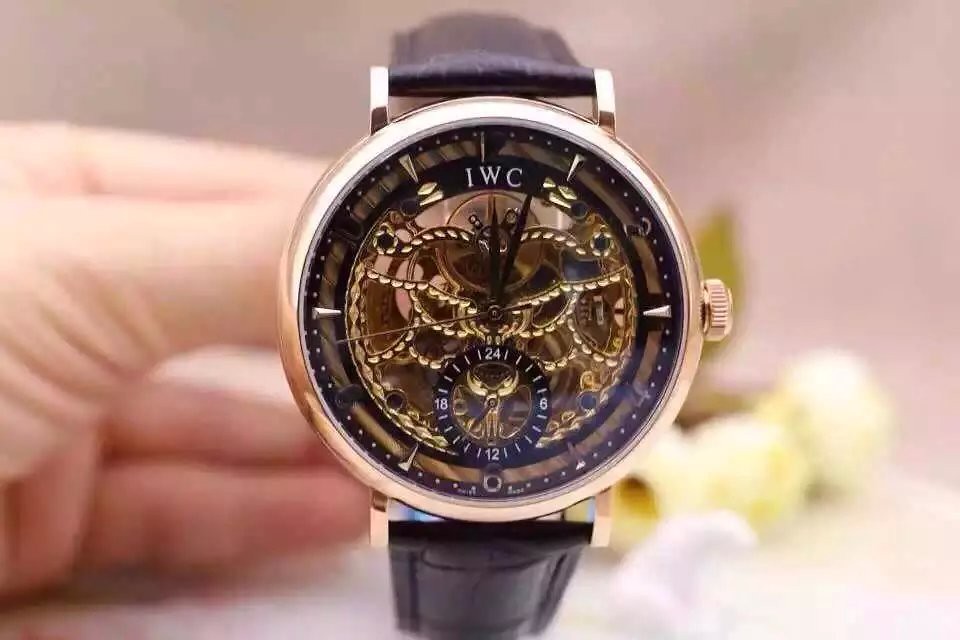This horizontally-oriented photograph features a left hand gently holding an elegant IWC dress watch. The hand is resting on an unseen surface, with the thumb and index finger delicately gripping the back part of the watch band, while the bottom two fingers hover just above the surface. The watch boasts an open-face design revealing its intricate inner mechanisms. Encased in a gold outer circle, the timepiece exudes luxury. The band is a rich dark navy, almost black, complementing the similarly colored outer rim of the dial and the watch hands. A secondary sub-dial positioned at the bottom displays the numbers 6, 12, 18, and 24 along its edge. The main watch face uses minimalist indicators at key points like three o'clock and nine o'clock, eschewing traditional numbers for a sleek, modern look.